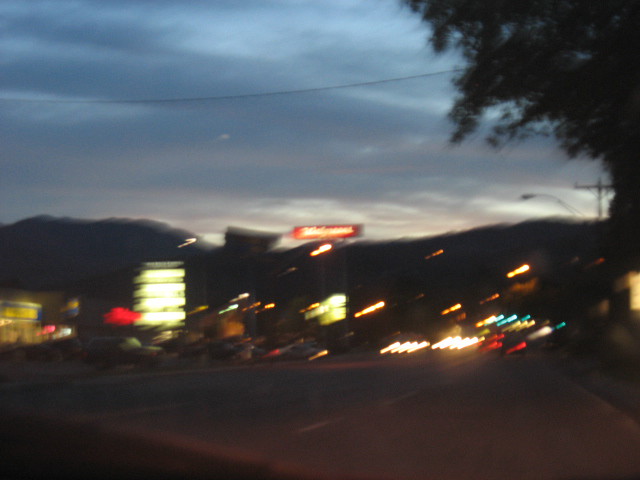An impressionistic view of a bustling street at dusk, captured from a moving vehicle. The horizon retains a hint of twilight, framing silhouetted mountains under a fading sky. In the upper right, a lone tree stands sentinel, while a power line stretches across the frame, adding to the scene's transient energy. The blurred image reflects the passage of time, with the taillights of cars ahead and the headlights of approaching vehicles. To the side, a shopping plaza with indistinct storefronts and illuminated signs glows faintly, contrasted by the soft blur of parked cars. The entire composition is a testament to the fleeting, dreamlike quality of a moment in transit.